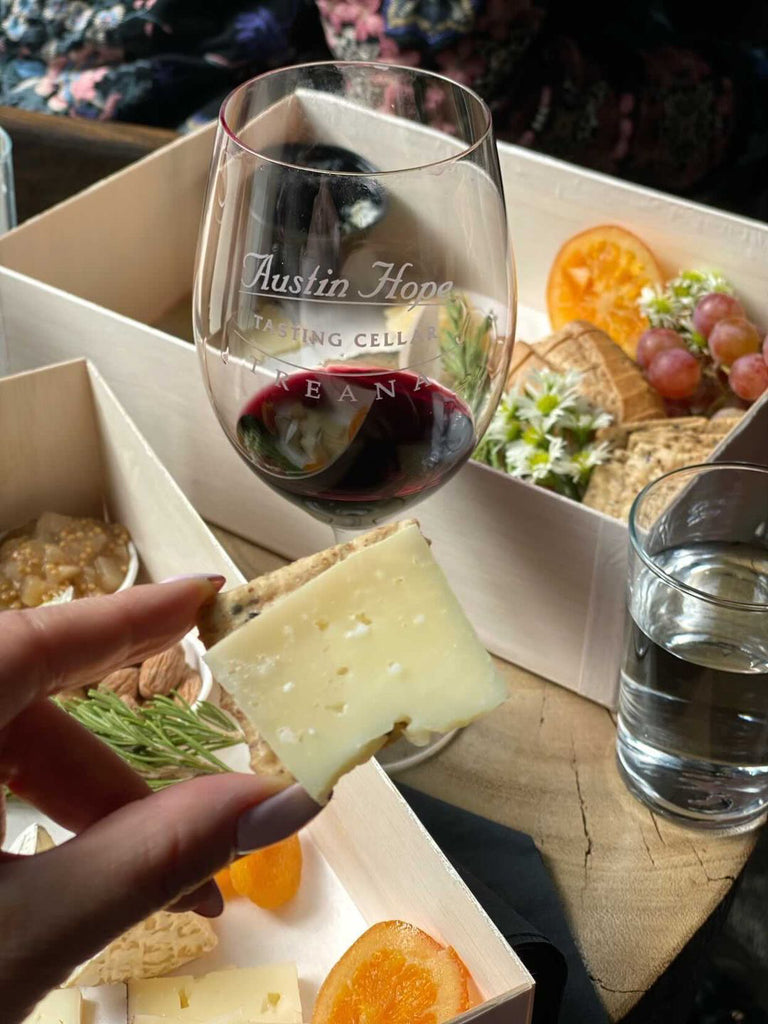The image captures a detailed close-up of a round wooden table set for a sophisticated wine tasting and charcuterie experience. The table, marked with characterful cracks, holds two open, rectangular, white pine-colored boxes filled with an assortment of gourmet treats. Inside the boxes, there's an enticing array of fruits including citrus slices and bunches of small grapes, rustic artisan bread, almonds in a small white porcelain dish, slices of pale butter-colored cheese with holes, and some chutney served in a white dish. Sprigs of fresh rosemary and thyme add a fragrant touch to the display. 

On the table, prominently displayed, is a glass of red wine inscribed with "Austin Hope Tasting Cellar." Near the wine glass, almost off the table's edge, sits a three-fourths-full glass of water, presumably for palate cleansing between tastings. The focus also includes a manicured hand holding a half-eaten cracker topped with a slice of cheese, positioned elegantly in front of the wine glass, partially obscuring its stem. The scene beautifully combines elements of indulgence, from the carefully curated charcuterie to the delicate tasting of fine wine, encapsulating a moment of refined sensory enjoyment.